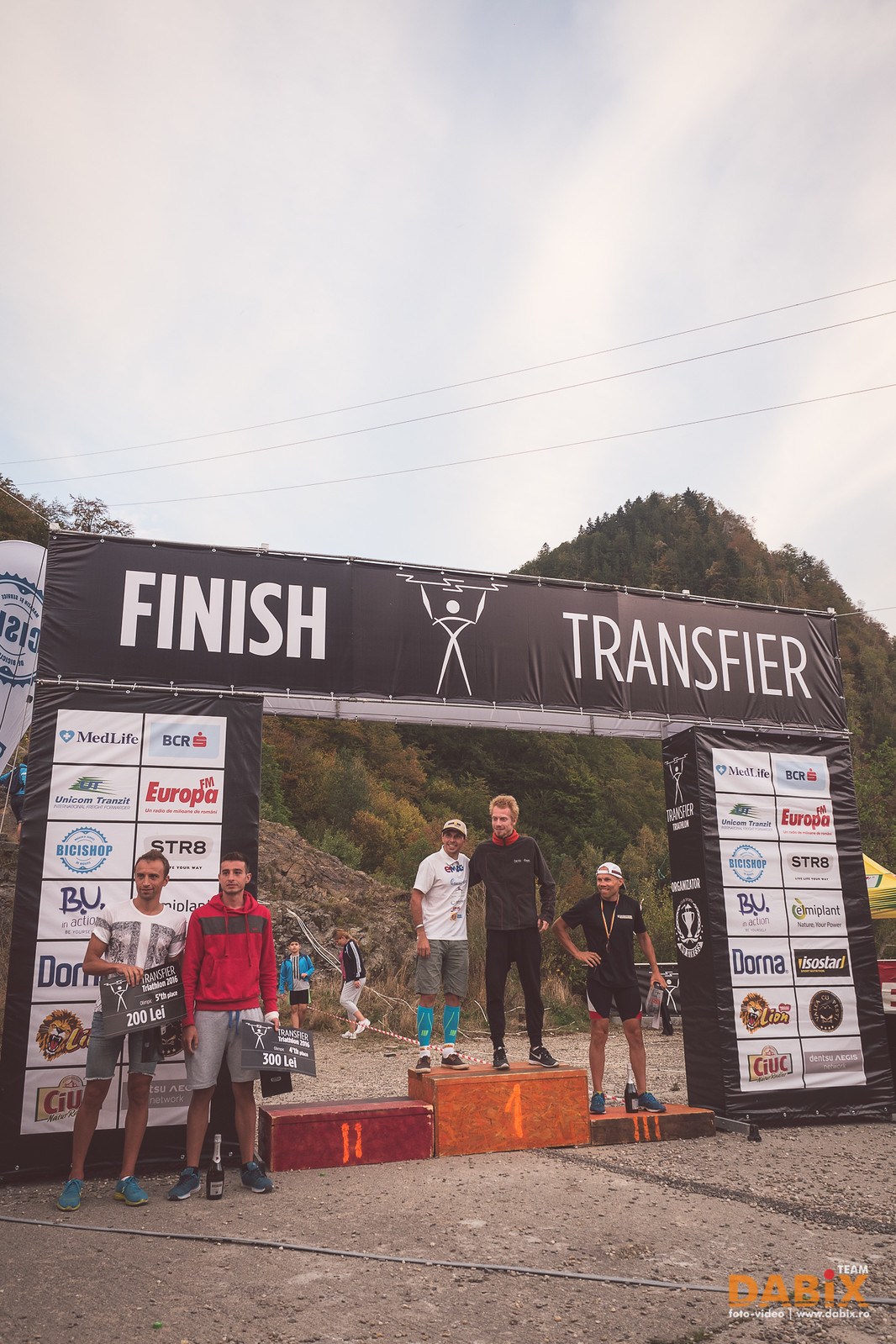The photograph captures a vibrant scene at an outdoor race event, set against a picturesque backdrop of lush hills with patches of brown and yellow hues. At the center of the image is a large winner's podium framed by a gate adorned with the words "Finish, Transfer." The podium itself is divided into three blocks, ascending in size from right to left, representing the 3rd, 2nd, and 1st places, respectively. Standing triumphantly on the largest block marked "1" are two men: one dressed in a black long-sleeve shirt and black pants, and the other in a white shirt with gray shorts. On the smallest block marked "3" is another man, wearing a white shirt and black shorts. The second place block is notably vacant.

To the left of the podium, two additional men stand holding signs displaying "200 LEI" and "300 LEI". One is clad in a red hooded sweatshirt and gray shorts, while the other wears a white shirt with gray shorts. The scene is set on a dirt floor amidst various sponsorship logos displayed on the columns around the podium, featuring brands such as MetLife and others in non-English script. A cartoon character logo is also prominently displayed at the top center of the scaffold surrounding the podium. The overall atmosphere of the image is celebratory, with the participants appearing happy and proud as they pose for the photograph.